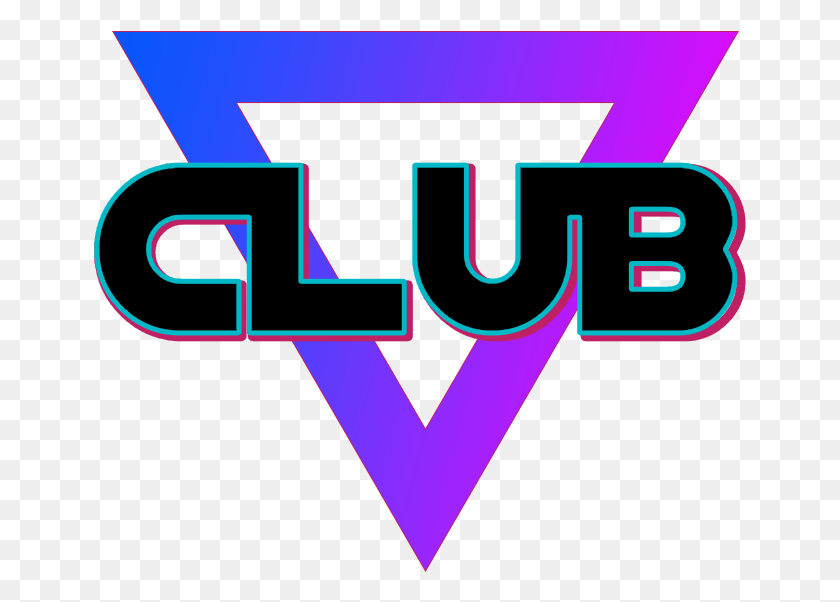The image features a retro, neon-inspired logo prominently displaying the word "CLUB" in the center. The background consists of a repeating pattern of small, white and gray checkered squares, often used for cropping or Photoshop backgrounds. The focal point is an upside-down triangle with a vibrant gradient shading: dark blue in the top left, pink in the top right, and purple at the bottom, with the colors smoothly transitioning into each other.

The word "CLUB" is layered over the triangle and designed with unique, connected scripting. The letters are black with a blue border and blend into each other; the top curve of the 'C' joins with the vertical line of the 'L', and the right side of 'U' merges into the top of the 'B'. The text also features a light purple drop shadow, enhancing its neon glow effect.